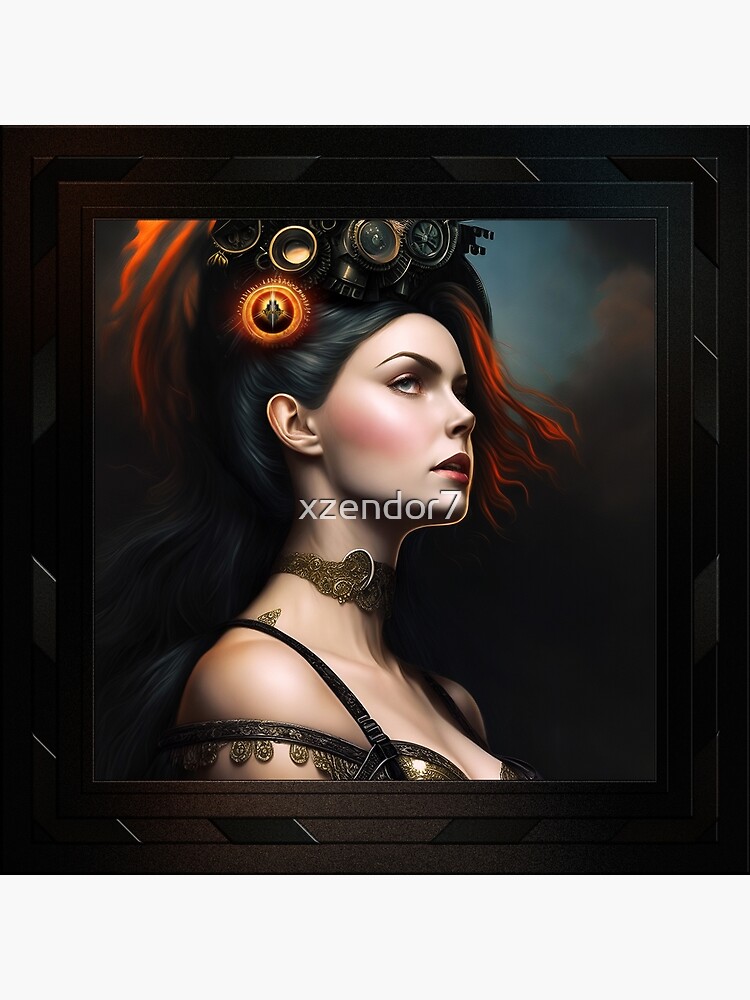The image portrays a digitally or AI-generated illustration of a young woman with fair skin and vibrant red lipstick, complemented by blush on her cheeks. She has long black hair, accented with striking red highlights, styled to hang well below her shoulders while a significant portion is artfully piled atop her head. This intricate updo is adorned with various metallic components, including lenses, timepieces, and a striking bright orange-yellow emblem resembling an explosion. The headwear features a steampunk aesthetic, incorporating elements of copper and dark brown metal. The background is a blend of dark gray and light blue with darkish white clouds, contributing to a mysterious atmosphere.

Around her neck, she sports a wide metal neckband with intricate gold inlays, adding a touch of elegance. Her attire includes a metallic bra made from gold-plated material and black leather, held in place with leather shoulder straps and an additional strap encircling her upper arm. The overall outfit exudes a fusion of futuristic and vintage styles, creating a captivating and intricate visual impression. The image is framed with what appears to be a wooden structure, possibly embedded with trapezoid-shaped rocks, further enhancing the unique and elaborate presentation.